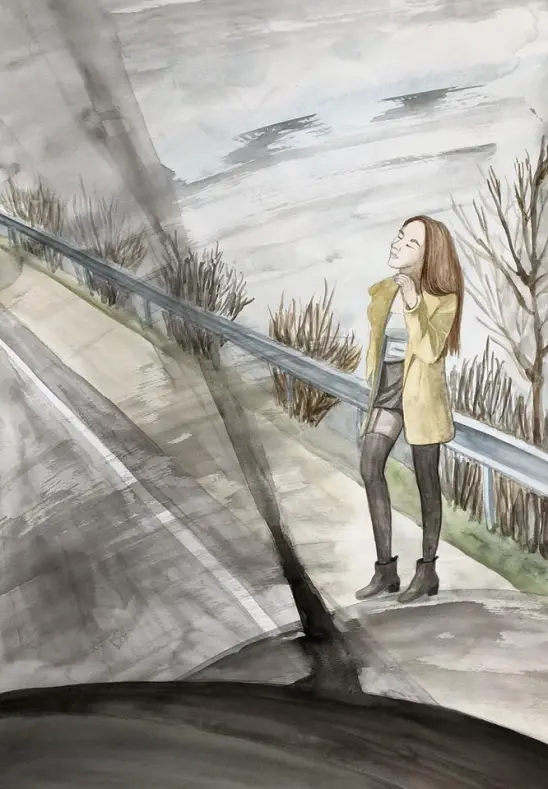This watercolor painting depicts a woman standing by the side of a busy highway, positioned against a metal guardrail. The perspective appears to be from inside a vehicle, looking out through a slightly blurry window. The woman, who seems to be hitchhiking, is wearing a yellow long-sleeve coat that is open in the middle, revealing a white t-shirt underneath. She is also dressed in a high-waisted short black skirt and tall knee-high black stockings, paired with black ankle-high booty heels. Her long brown hair cascades around her face, which is slightly tilted to the side with her eyes shut and her left arm raised towards her face. The background features a drab, gray, and faded sky with barren trees, indicating a winter scene. The painting's overall style is somewhat abstract and romantic, with the background appearing blurry and detailed only by brush strokes, enhancing the melancholic and introspective mood of the scene.